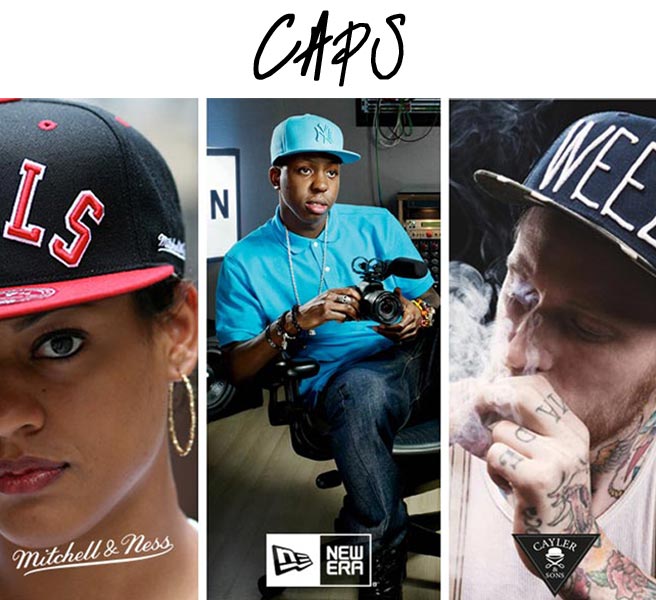The image features three vertical photographs showcasing individuals wearing different baseball caps, alongside the word "CAPS" in a unique uppercase font at the top of the image. 

- The first photograph on the left shows a close-up of an African-American woman wearing a black Chicago Bulls hat with red accents. She sports a gold hoop earring and the logo "Mitchell & Ness" is visible at the bottom of the image.
  
- The middle photograph depicts an African-American man seated in a black desk chair, set in a gray-walled room. He is wearing a blue polo shirt, blue jeans, a blue Yankees cap by New Era, and a long necklace. A TV is visible behind him, suggesting he might be in a recording studio or home office.
  
- The photograph on the right features a man with tattoos on his neck, arms, and hands. He is wearing a black hat that reads "Weed" and a white shirt, smoking something that emits visible smoke. The logo "Kaler" appears at the bottom of this image.

The image highlights a diverse array of individuals and styles, emphasizing different brands and types of caps through a comparative display.